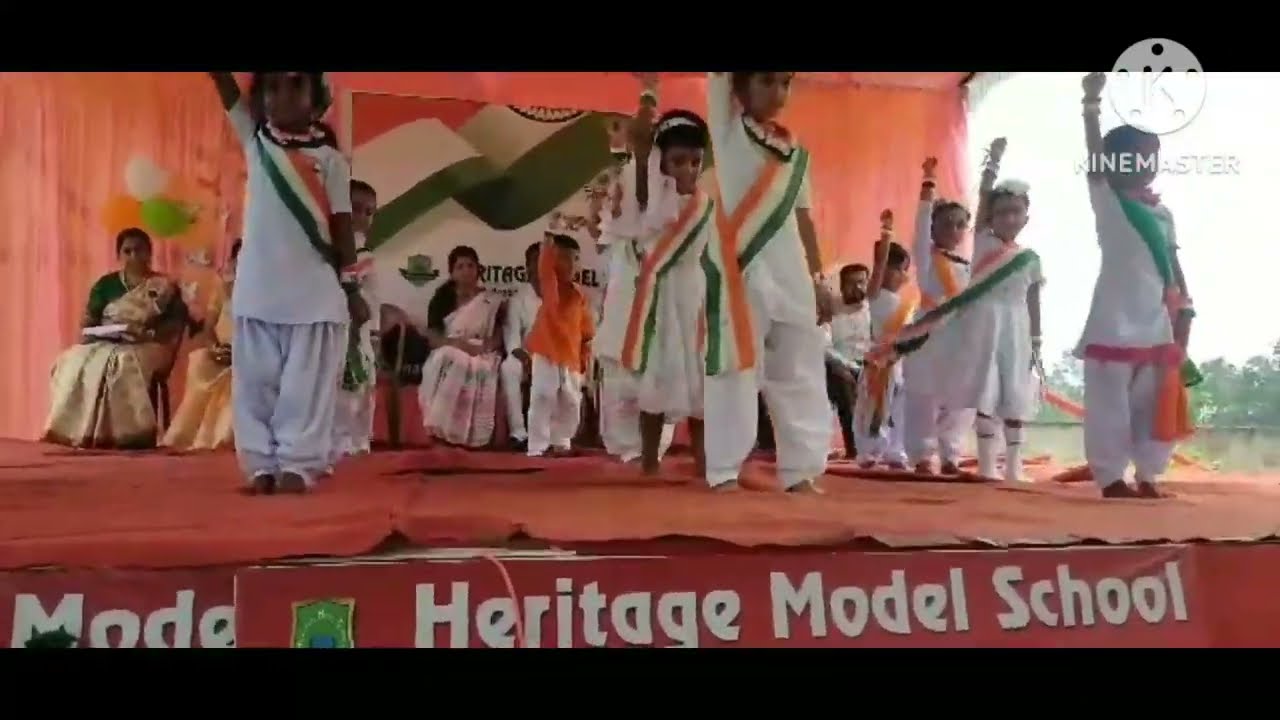The image depicts an outdoor ceremony or performance at the Heritage Model School, as indicated by the white text on the orange stage. Central to the photo, a group of children, comprising both girls and boys, stand barefoot in three columns with their fists raised in a defiant posture. Each child is dressed in white clothing—shirts and pants—and adorned with sashes featuring the tri-color scheme of the Indian flag: orange, white, and green. Surrounding the children, a group of teachers or adults sits watching attentively. The stage itself is vibrant with an orange carpet and matching curtains, while the background includes a large, prominently displayed flag. To the right, past the stage, trees and a bright sky are visible, indicating the event is taking place outdoors. Additionally, a logo with the letter 'K' for KineMaster and the word 'KineMaster' appears in the upper right corner, suggesting that this might be a still from a video.